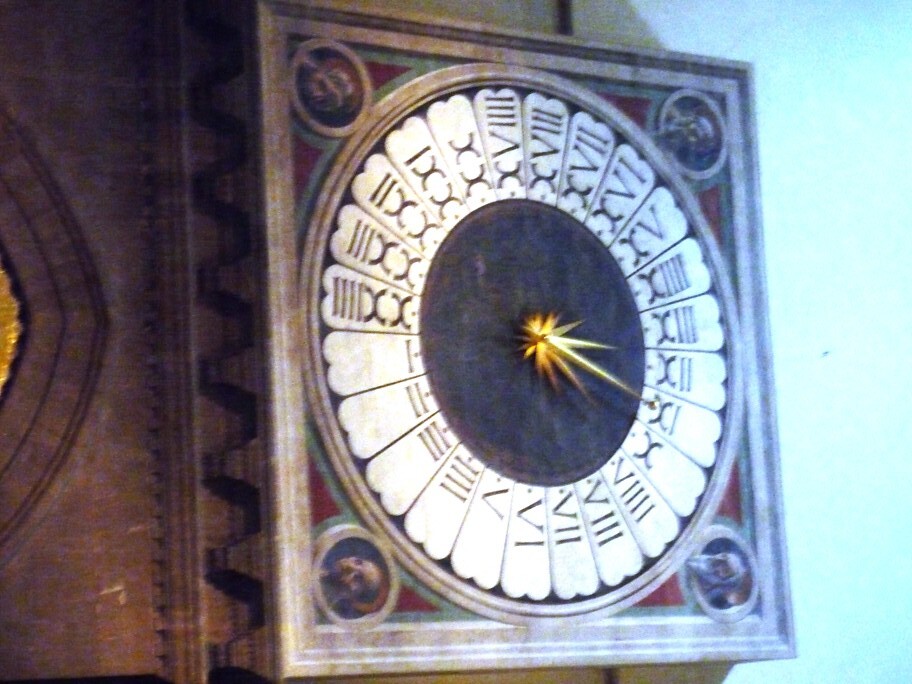The image depicts an antique, 24-hour analog clock with a unique and distinctive design. The clock is presented at a sideways orientation, making the faces of bearded men in the four corners appear tilted and slightly blurred. The clock’s face features Roman numerals arranged in segments resembling pie pieces, numbered sequentially from 1 to 24. Notably, the clock has a striking central design element: an hour and minute hand that both resemble a sunburst or explosion extending outward. The surrounding structure of the clock seems to be made of wood, enhancing its vintage appeal. The clock, set against a backdrop where the ceiling appears to the right and the base to the left, suggests an image taken from an unusual angle, further emphasizing its old-fashioned, perhaps even antique, character.